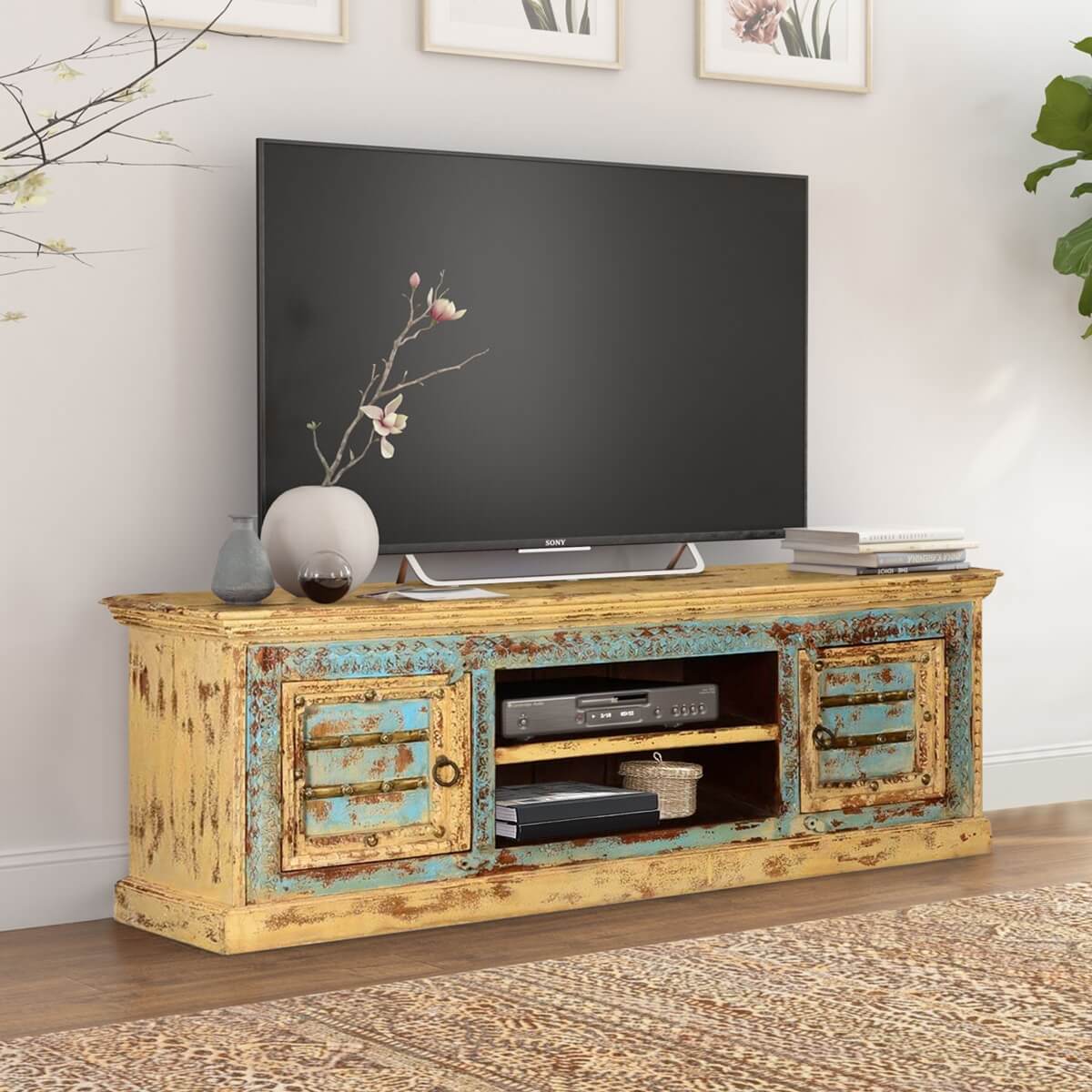The professionally photographed image showcases a living room with a modern large-screen Sony TV set atop a long, distressed media center. The TV, sleek and black, contrasts starkly with the aged look of the TV stand, which appears to have been originally brown but deliberately painted with yellow-tan and light blue hues, then distressed to reveal patches of the underlying color, giving it a rustic, worn-out look. The media center features two closed drawers on either side, with a middle section housing a DVD player, two books, and a small basket. To the right of the TV are a stack of three or four books and a box similar to a hat box. On the left side of the media center, there are three decorative vases: a blue vase, a smaller liquid-filled sphere, and a larger white sphere vase holding two white and pink flowers with one bud. Above the setup hang three floral paintings, prominently featuring a pink flower. Just visible at the edges of the image are two decorative plants, one lush with leaves and the other bare. The setting includes a white wall, a wooden floor, and a tan-brown carpet placed in front of the media center.